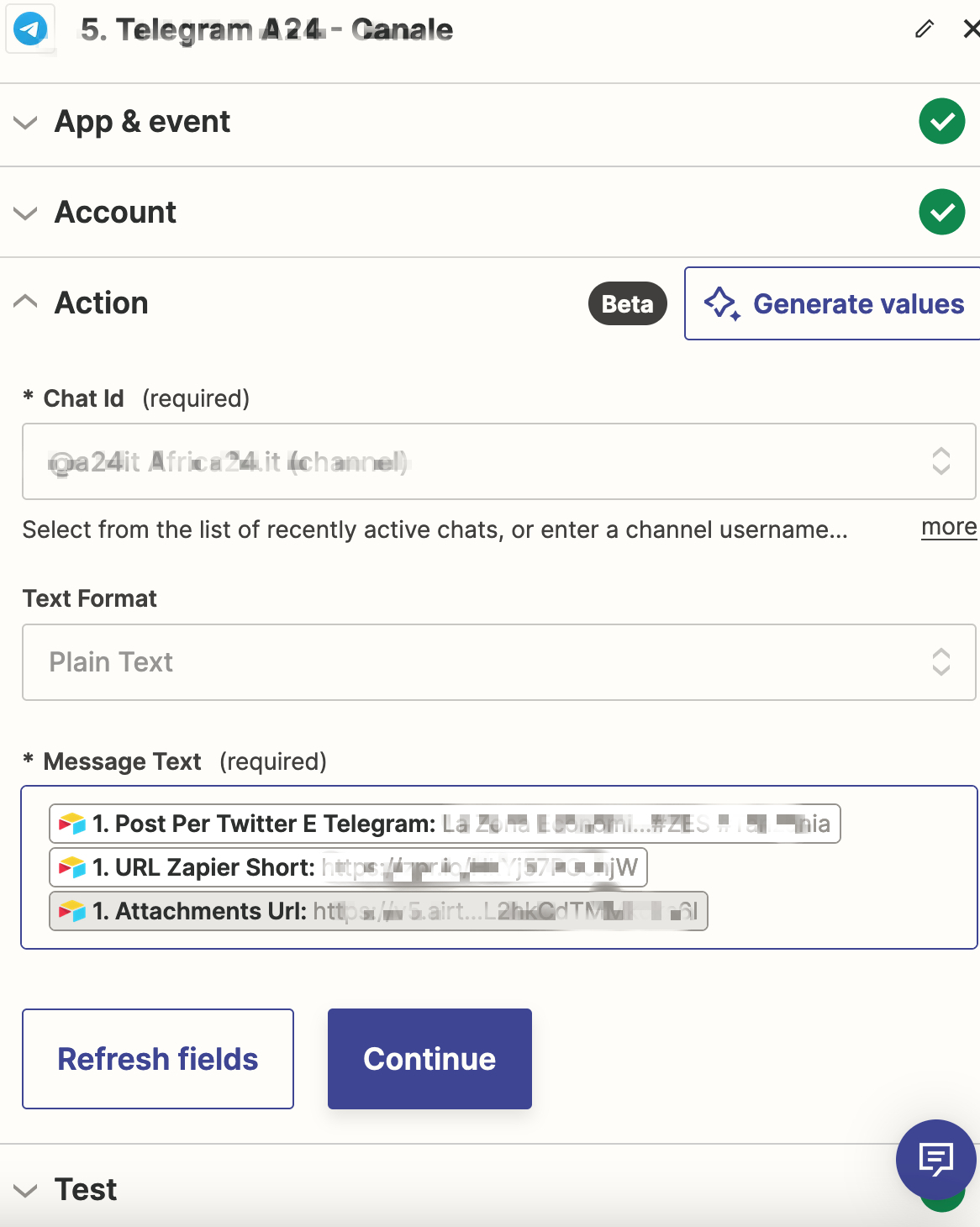A screenshot of a form being filled out within a web application. The interface features a blue circle and a gray square icon, resembling a paper airplane pointing northeast, indicative of a messaging service. Prominently displayed is the label "Telegram" at position number five, accompanied by some symbols and the name "Ganali." The text appears in a gradient from dark gray to black, suggesting a typewriter-like font that's running low on ink. 

At the top, there's an option for users to draw or write on the form, marked with an X. Below it, there's a drop-down menu titled "App and Event" with a green check mark, indicating a valid selection. Adjacent to this is another drop-down menu labeled "Account," also marked with a green check. 

The section titled "Action" is expanded and marked as "beta." It includes fields where users can "generate values," input a "chat ID," and select from a list of recently active chats or enter a channel username. Plain text instructions are provided, followed by a list of three message texts: "posts per Twitter e-telegram," "URLs," "Zapier," and "Short," with associated attachment URLs.

At the bottom, there are two buttons—a white "Refresh Fields" button and a blue "Continue" button—allowing users to update or proceed with the form.